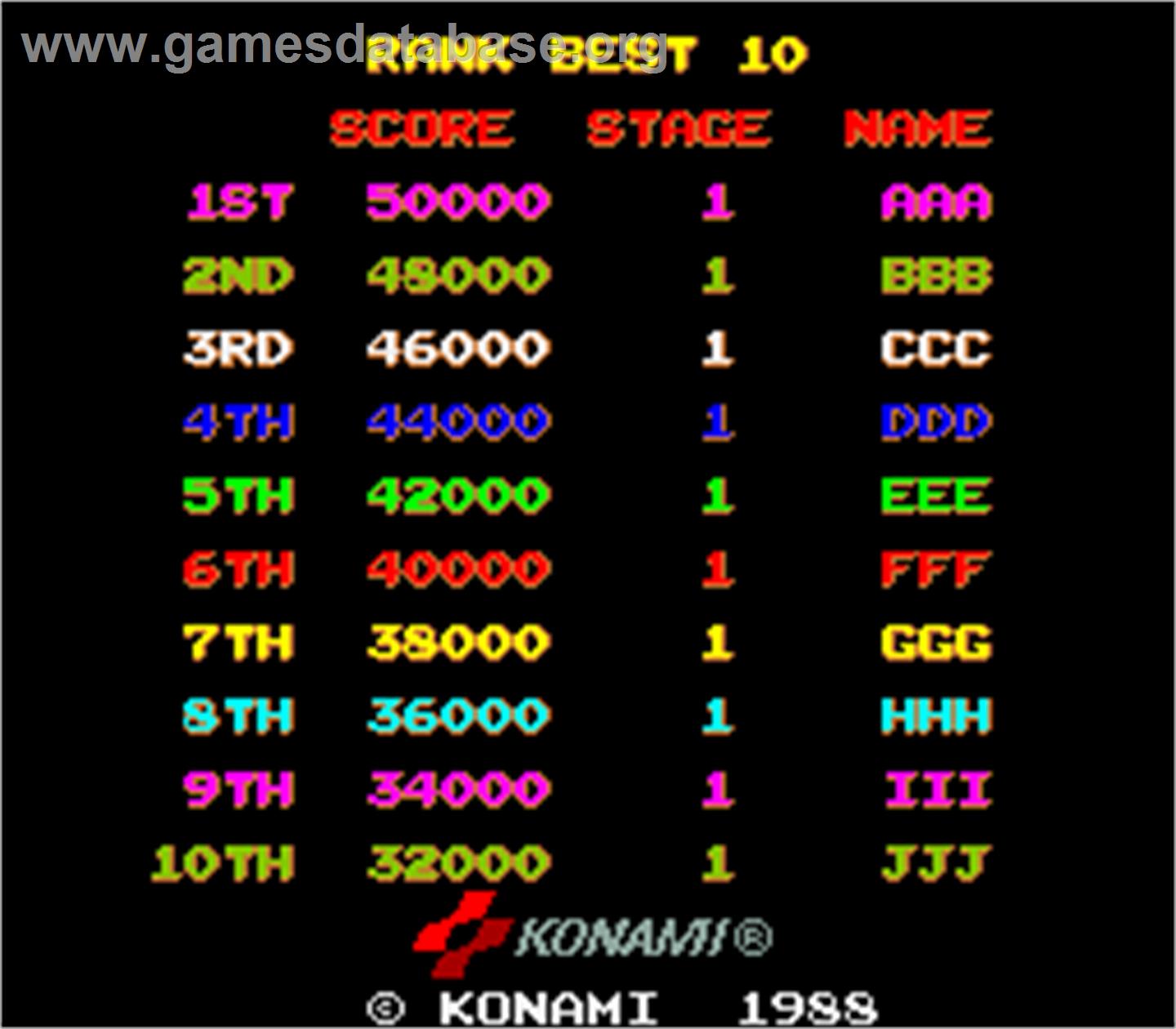The image depicts an old video game scoreboard set against a black background. At the top, a partially legible translucent watermark reads "www.gamesdatabase.org," overlaying the yellow text "RANK BEST 10." Below this, in red lettering, it states "SCORE," "STAGE," and "NAME." The scoreboard lists the top ten scores, displaying a diverse array of colors: pink, green, white, blue, bright green, red, yellow, light blue, pink again, and light green. The scores range from 50,000 to 32,000, with all entries marked under "Stage 1." Each score is associated with a three-letter initial, from AAA to JJJ. At the bottom center, the image features the Konami logo with a red and dark red swoosh design, and the text "Konami" alongside "© Konami 1988."